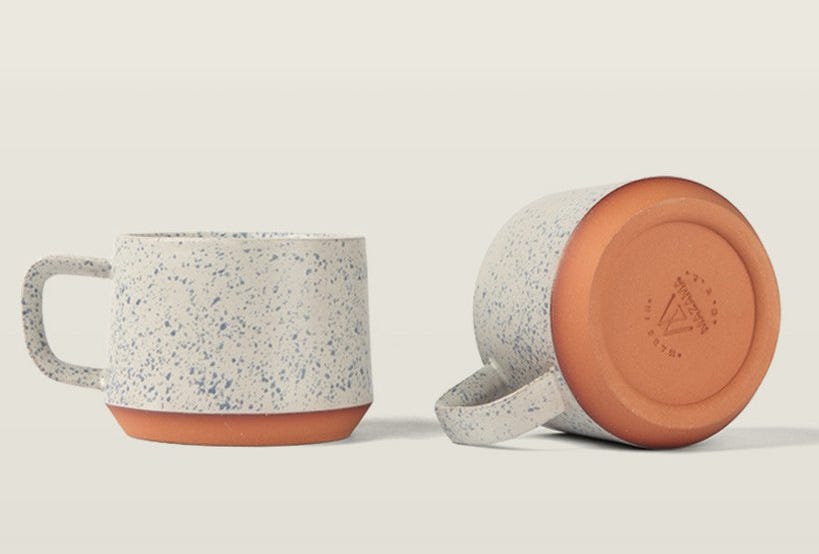This image depicts two stoneware coffee mugs set against a completely white background. Both mugs feature a cream-colored base with blue speckles, evoking a camping style aesthetic. One mug is positioned flat on the surface with its handle pointing to the left, hiding its bottom inscription. The other mug lies on its side with its terracotta-colored bottom in clear view, revealing the etching "M-A-Z-A-M-A" along with an "M" logo inscribed into the base. The overturned mug's handle, which also points left, touches the white surface, emphasizing its geometric contours. Shadows fall to the right of both mugs, enhancing the minimalistic yet detailed composition of the scene.